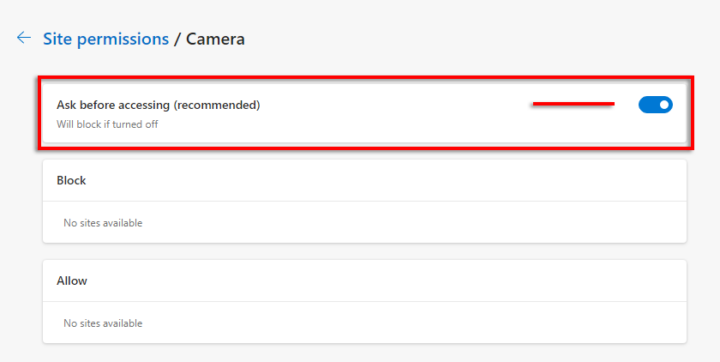The image displays the "Camera" section within the "Site Permissions" settings of a computer. The interface features a predominantly white background, except for the "Site Permissions" and "Back" buttons, which are highlighted in blue. The "Camera" section is prominently displayed in black text, as are the other explanatory texts within the section.

Within the "Camera" settings, there are three options available for user selection. The first option is "Ask before accessing (recommended)," which is currently highlighted and selected by the user. This option is indicated by a red square around it and a blue slider toggled to the 'on' position, signifying the user's preference to be asked before any website gains camera access.

The second option is "Block," under which no sites are listed, indicating that the user has not blocked any sites from accessing the camera. The section appears as an empty white square.

The third option is "Allow," and similarly, it shows "No sites available," meaning the user has not pre-approved any sites for camera access.

Overall, the user has configured the settings to ensure the camera access is regulated by confirming permission for each site individually, thereby preventing automatic activation of the camera without the user’s explicit consent.